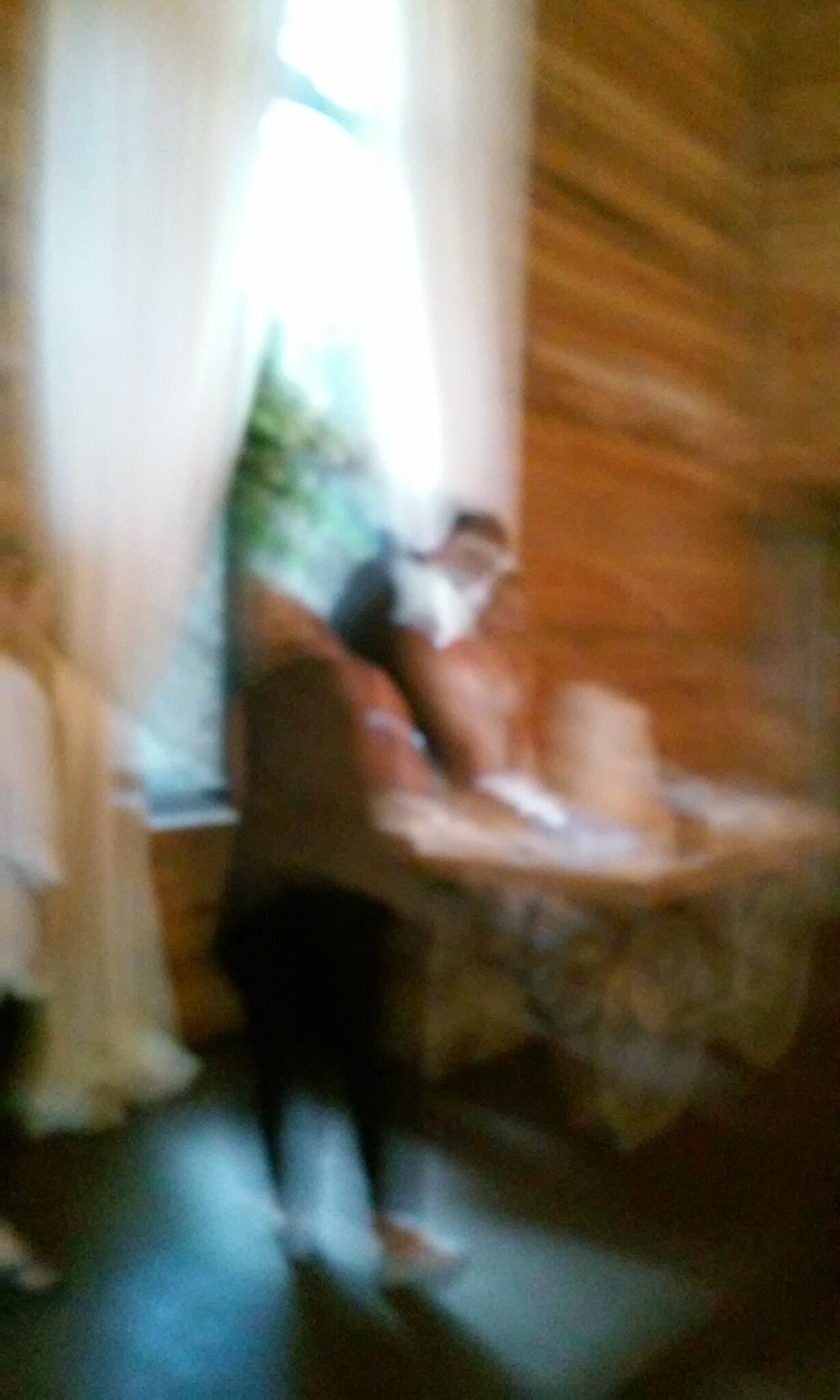In this extremely blurry indoor photograph, taken at standard eye level and slightly upwards, the foreground features a person walking towards an old-style flat cart table with large spoked wooden wheels. The person, dressed in black pants, a pink or tan shirt, and white sneakers, is navigating a darker-colored floor. Positioned centrally, the left side of the frame is dominated by a large vertical window dressed in white sheers, through which filtered sunlight and out-of-focus trees are visible. In front of the window, two or three individuals stand, highly blurred, with one possibly being a bride in a white wedding dress and another potentially a groom. On the table, a multi-layered wedding cake is discernible. The background wall on the right side of the frame is constructed from horizontal wooden panels or possibly logs, contributing to the rich, grainy texture of the image. The entire scene is brightly lit but extremely out of focus, rendering all subjects and objects indistinct.